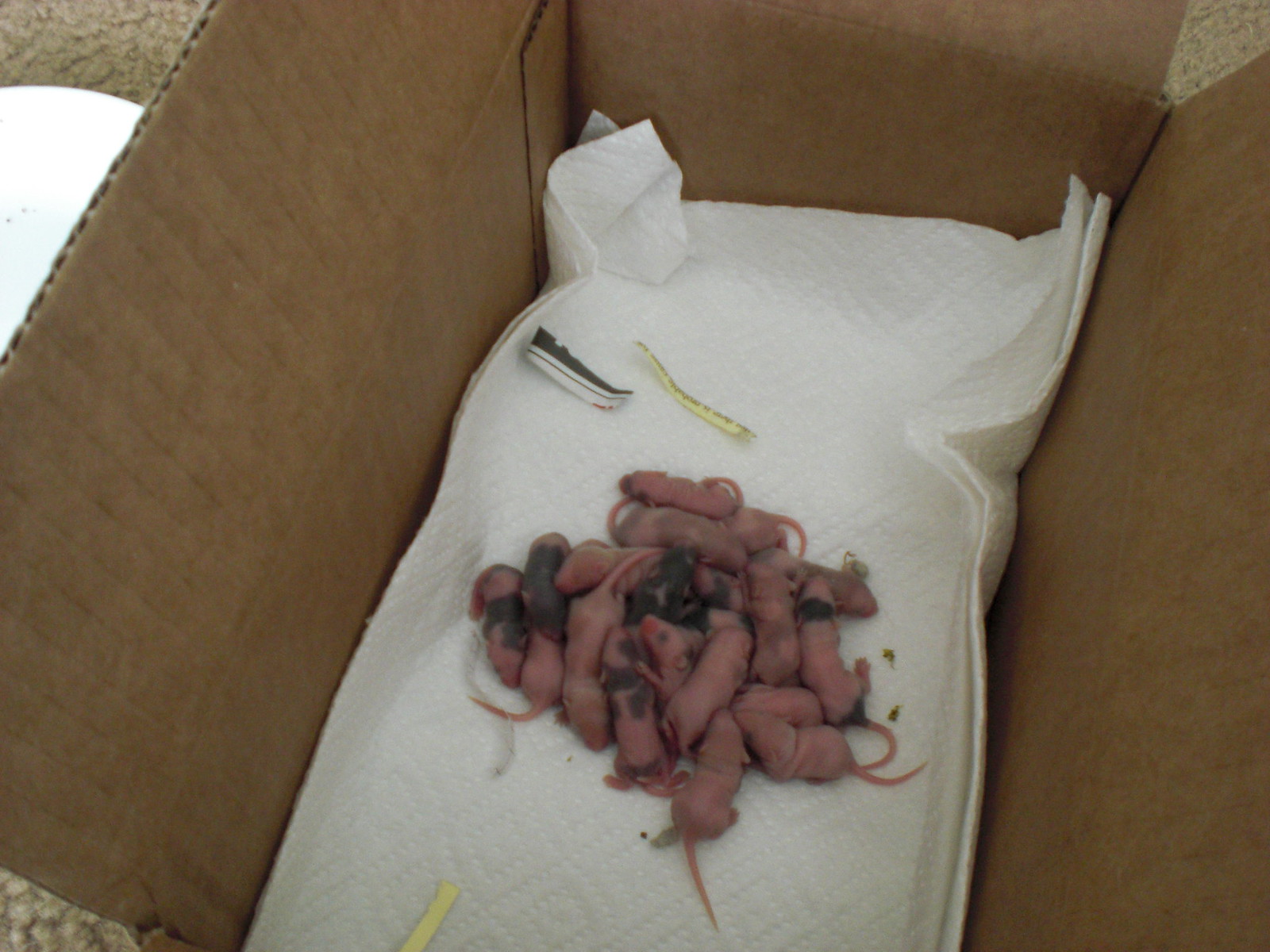The photograph depicts a close-up view inside a large, deep, tan cardboard box, revealing a pile of baby rodents, possibly mice or rats, although the exact species is uncertain. These newborns, numbering at least between 12 and 20, are predominantly pink with some black and gray spotting, and they are hairless, flaunting their underdeveloped eyes, small paws, tiny feet, and long tails. They are huddled together, positioned centrally on top of white paper towels that cover the bottom of the box. Scattered around them are shredded pieces of yellow and black-striped newspaper and tiny feces. The cardboard box, lined with paper towels, sits on a carpeted floor, adding a layer of context to the environment. The overall appearance suggests the image might be slightly older and not of the highest quality, contributing to its raw, intimate depiction of these vulnerable, very young animals.